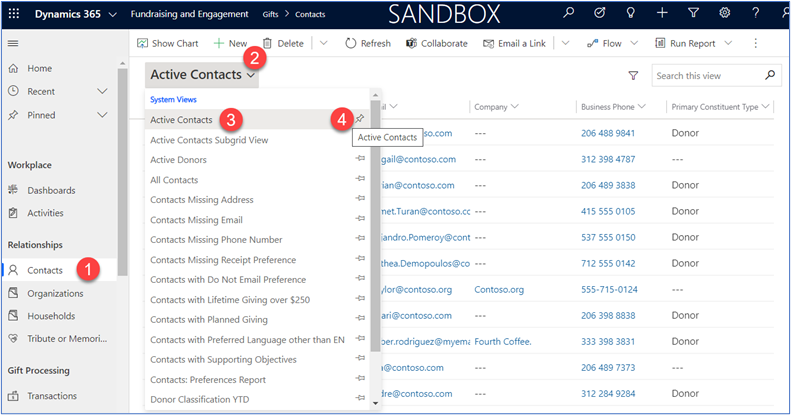This image is a screenshot from the Dynamic365 website, specifically showcasing their Fundraising and Engagement module. The interface prominently displays the word "SANDBOX" in capital white letters centered at the top within a black rectangular header. Along the left side, the background transitions from black to gray, while the central area is predominantly white. Blue text appears in several places within the white background, including a notable "System Views" label.

The screenshot also features four numbered markers within red circles. 

1. Number 1 is adjacent to the "Contacts" section.
2. Number 2 is positioned higher on the screen near the "Active Contacts" section.
3. Number 3 appears slightly lower and also corresponds to the "Active Contacts" section.
4. Number 4 is situated near an icon and close to the previous marker.

Most of the remaining text on the screen is in black or gray, providing clear contrast against the varying background shades.